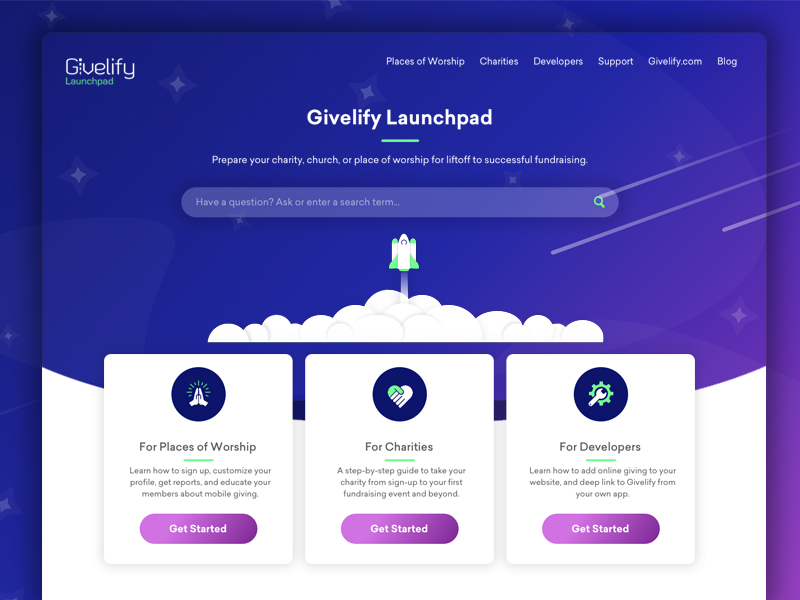This image is a cropped snapshot of the homepage for the Give Lifey website. 

At the top left corner, the Give Lifey logo is prominently displayed with the words "Give Lifey Launchpad" next to it, with "Launchpad" highlighted in green. 

On the top right side, there is a navigation menu in small white font listing the following categories: Places of Worship, Charities, Developers, Support, GiveLifey.com, and Blog. 

Centralized at the top of the page, “Give Lifey Launchpad” is written, with a small green horizontal line directly below it. Beneath this line, a tagline in small white letters reads, "Prepare your charity, church, or place of worship for liftoff to successful fundraising." 

Directly below this tagline is a prominently centered, long search bar. 

Just beneath the search bar, there is a graphic illustration showcasing a spaceship lifting off above the clouds. 

Below the graphic, three white boxes are centered on the page:

- The first box on the left is titled "For Places of Worship," followed by a brief description and a purple "Get Started" button at the bottom.
- The middle box is labeled "For Charities," also accompanied by a short description.
- The third box on the right is labeled "For Developers."

This layout is visually designed to guide users towards their specific areas of interest for better engagement.